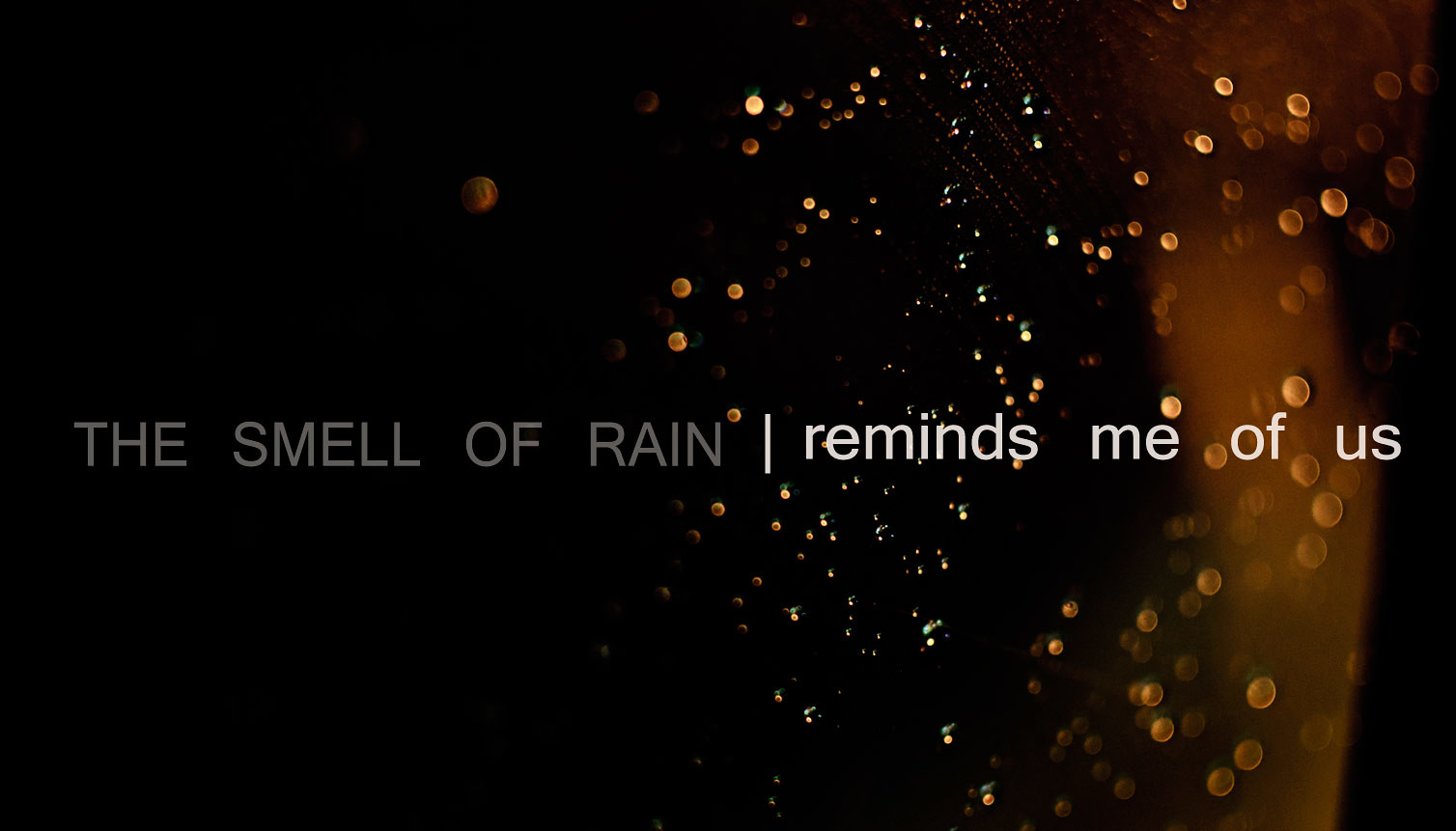The image features a minimalistic graphic design set against a black background with a striking array of varying-sized droplets, some clear while others glow with hints of amber and white hues. These droplets resemble rain splashes, artfully scattered as if clinging to a window. Running horizontally across the center of the image is a poignant message rendered in all caps; the gray text "THE SMELL OF RAIN" on the left, separated by a vertical white line, transitions into white text stating "REMINDS ME OF US" on the right. This thoughtful composition evokes a nostalgic connection to rainy moments shared.